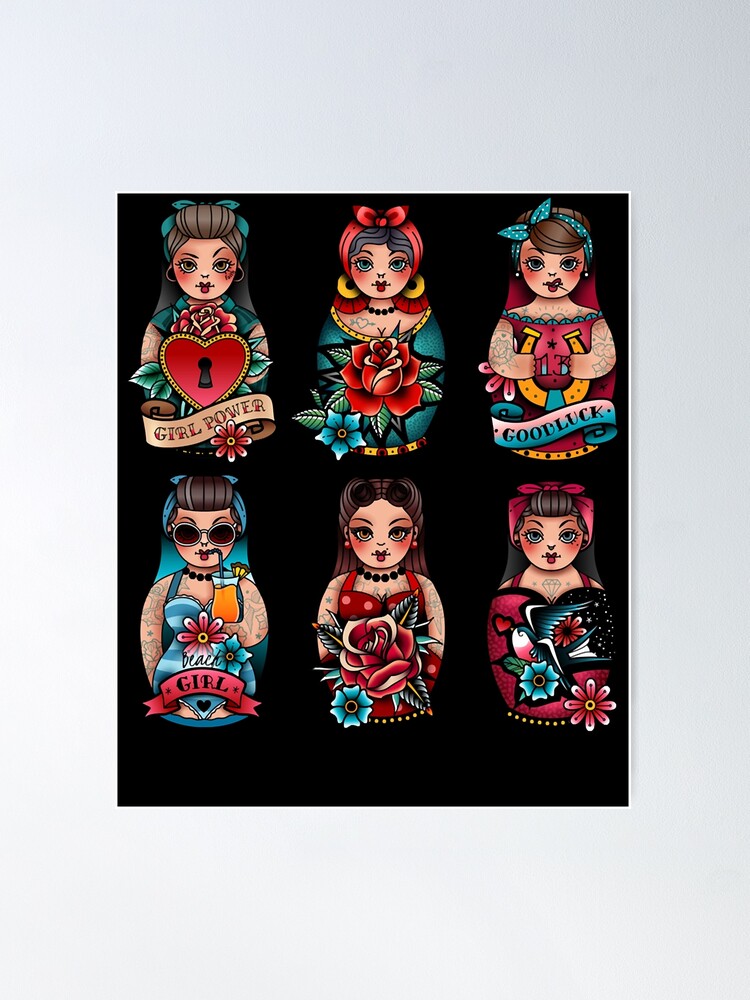The image displays a set of six beautifully illustrated dolls, arranged in two rows of three, each embodying a vibrant, slightly whimsical character. Set against a stark black background framed by a delicate dark grey border, these dolls evoke the form of traditional Russian nesting dolls but are distinctly not in that style. Instead, each doll is designed in a cheerful and contemporary fashion, with a style reminiscent of digital or Mexican folk art, featuring rich hues of yellows, darker pinks, reds, and blues.

In the top row, starting from the left, the first doll is a light-skinned woman with gray hair tied up in an aqua bow. She is adorned with a red heart framed in gold and a banner beneath it reading "Girl Power." The middle doll of the top row holds a red rose and dons a vibrant red bandana, while the doll on the right showcases blue tattoos and a blue and white polka dot bandana, holding a yellow horseshoe near her face with a banner proclaiming "Good Luck."

On the bottom row, the leftmost doll is labeled "Beach Girl." This character is a light-skinned woman with a plethora of tattoos, wearing a blue-striped swimsuit, black hair tied in a blue bow, and brown sunglasses while sipping a tropical drink. The middle doll again holds a rose, and the one to the far right is adorned with an array of pink and blue flowers.

This collection of images, presented in a portrait orientation with a light gray outer frame, offers a striking and colorful visualization, each doll encapsulating a unique piece of affirmative art.